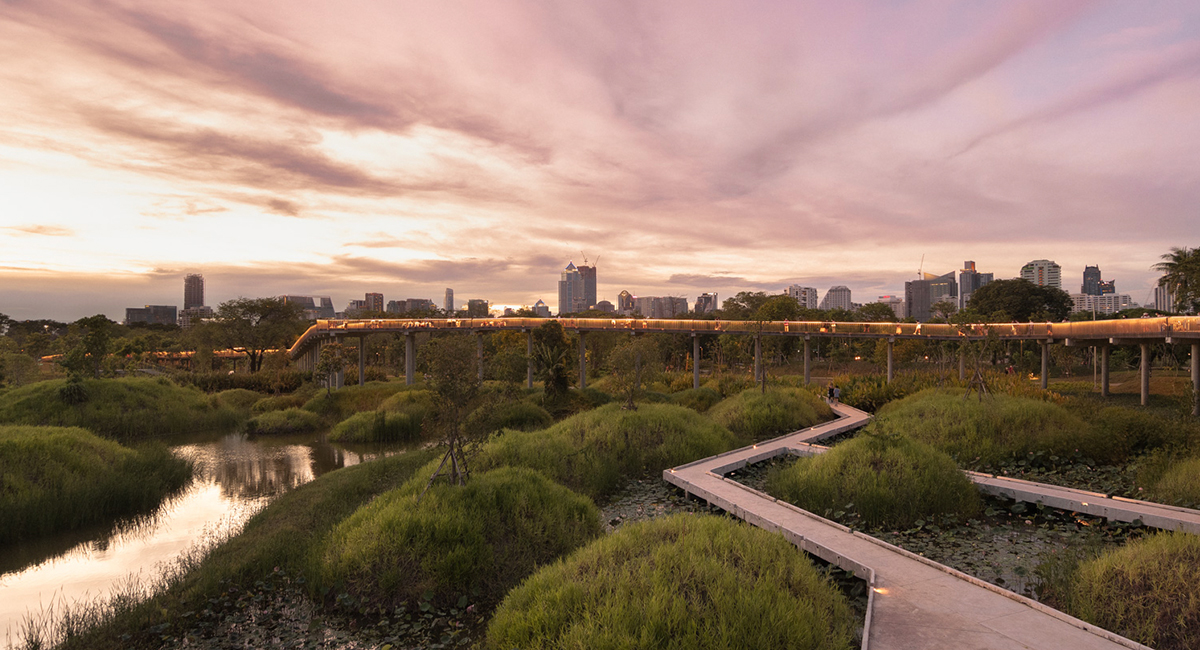In the image, a cityscape unfolds under a mesmerizing sunset sky that transitions from a warm peach yellow on the left to patches of pink and lavender tones on the right, all amid rippled clouds. At the horizon, clusters of tall buildings mark the city's skyline. Below them, a raised roadway or tram track, illuminated and supported by large concrete pylons, extends across the scene. In the foreground, on the bottom left, a small stream or stretch of water winds through green patches of hills. To the right, a wooden pathway resembling a dock navigates through the greenery and connects toward the roadside, lying beneath the raised roadway. The interplay of vivid sky colors and diverse structural elements creates a visually striking and detailed urban landscape.